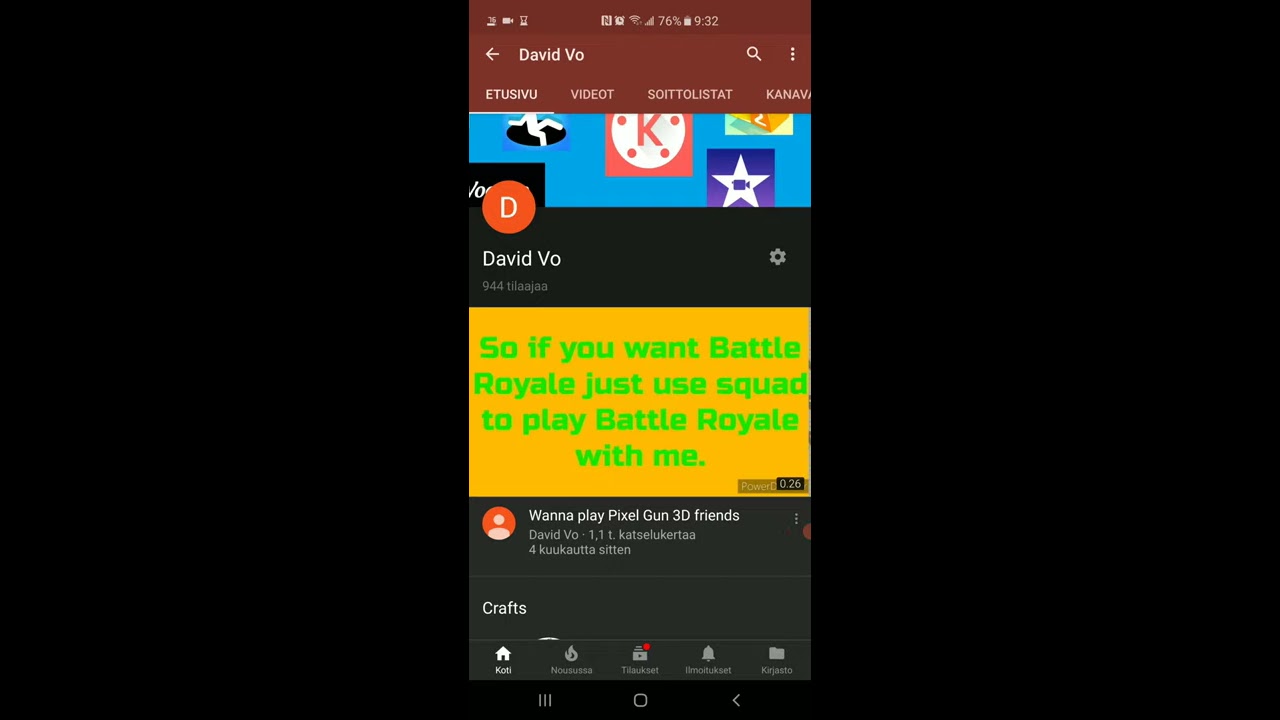This image is a detailed screenshot of a cell phone display, possibly an Android device, given the layout and design. The screen displays multiple elements in a mix of English and another language. The background is primarily burgundy, transitioning into blue and yellow sections, with blacked-out strips on either side, suggesting the image is narrower than the phone's full screen.

At the top, the phone's status bar reads "76% battery" and "9:32 AM" in white text. Below this, the name "David Vo" appears alongside a left-pointing arrow, a magnifying glass icon, and a hamburger menu icon, all in white. There is a series of non-English words: "ATUSIVU," "VIDEOT," "SÄKÄ LISTAT," and "KANAVA," also in white.

The main section of the image features a colorful collection of various logos and icons. There is a red circle with a 'K' in white, a star-shaped symbol with a blue camera, and a profile picture icon labeled "D" for David Vo. These are placed against a blue and gold backdrop that simulates a water effect. Another timestamp reads "9:44," followed by more text in an unfamiliar language, possibly denoting the user's current activities or notifications.

Prominently, there is a gold rectangle with green text that states, "So if you want Battle Royale, just use Squad to play Battle Royale with me." Below this, on a gray background, white text asks, "Wanna play Pixel Gun 3D Friends?" 

The bottom of the screenshot includes additional options and symbols like a settings icon, a small person in an orange circle, a flame symbol, folders, and a bell. Various white texts on black and gray backgrounds indicate interactive elements such as "Crafts," "Cool Cults," and navigation buttons like the hamburger menu and left arrow.

The visual palette of the screenshot includes colors like yellow, green, gold, red, pink, multiple shades of blue, maroon, black, white, and gray, making for a rich and diverse display. This meticulous composition of icons, text, and colors strongly suggests a screenshot from a YouTube application or a similar social media platform on David Vo's phone.